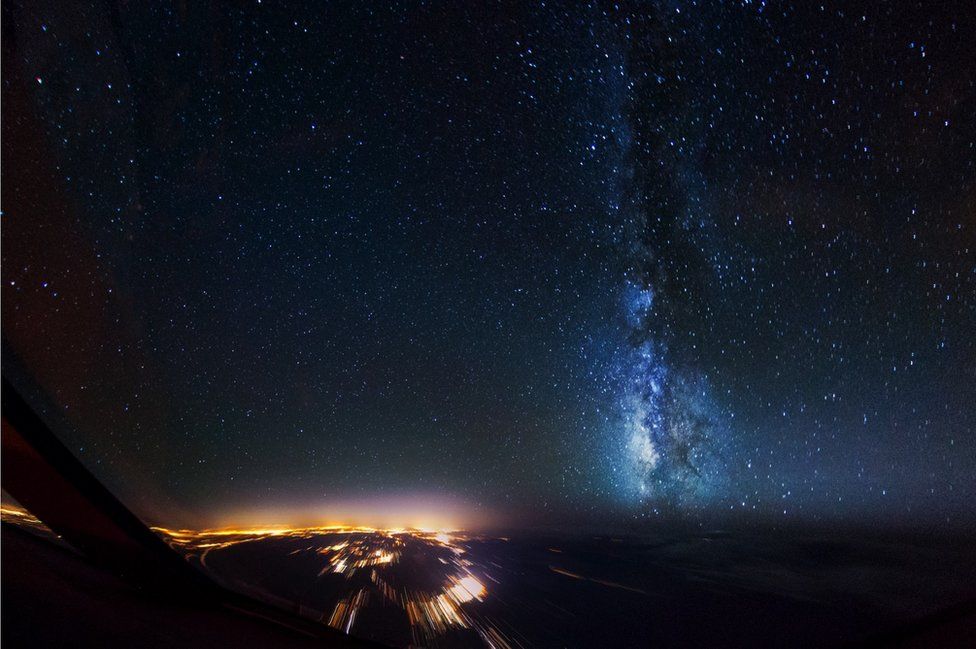This captivating image captured from a moving aircraft, possibly an airplane, helicopter, or spacecraft, showcases a stunning night sky filled with countless stars scattered across the dark blue to black expanse. Toward the right side, a mesmerizing cloudy mixture of blue stars, resembling a galaxy, adds depth and intrigue to the scene. The lower portion of the image features vibrant streaks of light from streetlights and city glow, illustrating the hustle and bustle far below. Near the bottom left corner, a part of the aircraft's frame is visible, grounding the viewer in the perspective of the photographer. Accentuating the bottom edge is an orangey hue that subtly transitions into the blackness below, possibly reflecting the distant city lights or the horizon. The overall effect is a well-lit, panoramic view that beautifully encapsulates both the serenity of the night sky and the lively sparkle of urban areas below.